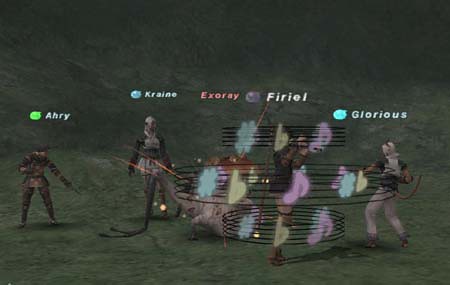The image appears to be a still from a video game, featuring a somewhat blurry digital graphic with a dark green background that resembles either a textured floor or grass. Five characters are visible on the screen, each with a unique name and colored dot above them. On the far left, there is a man dressed in a brown-black outfit with a black hat, named A-H-R-Y, with a green dot above his name. The next character is a bald man looking in the other direction, named Crane, highlighted by a blue dot. Moving right, is a figure named E-X-O-R-A-Y with a purple dot next to their name. F-I-R-I-E-L is the fourth character, marked by a blue sphere and surrounded by black swirls. Lastly, on the far right, there's G-L-O-R-I-O-U-S with a white sphere, dressed in a black top with white pants and possessing blonde hair. Overlaying some characters are musical notes on a circular grid, featuring notes in purple, green, and yellow, amid musical lines in black. A large animal figure is also positioned just behind these musical notes.